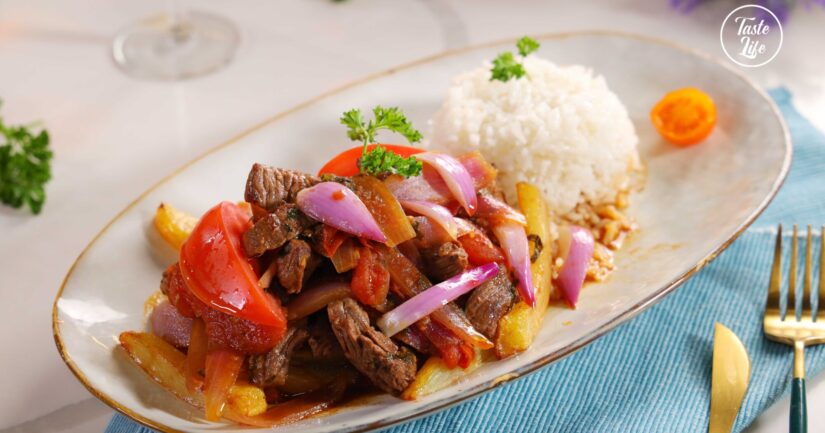The image features a long, oval-shaped white dish adorned with a gold trim, containing a stir-fry mixture of cut-up brown beef, red onions, red and orange peppers, interspersed with leafy green parsley. Adjacent to the stir-fry, on the right side of the dish, lies a scoop of white rice garnished with green leaves. The dish is set on a table draped with a blue and white napkin. Gold and black utensils – specifically a knife and a fork – are partially visible at the bottom right corner of the image. In the background, there's a clear wine glass and a white tablecloth covering part of the table. In the top right corner of the photo, a white circle contains the words "Taste Life" written in black text.